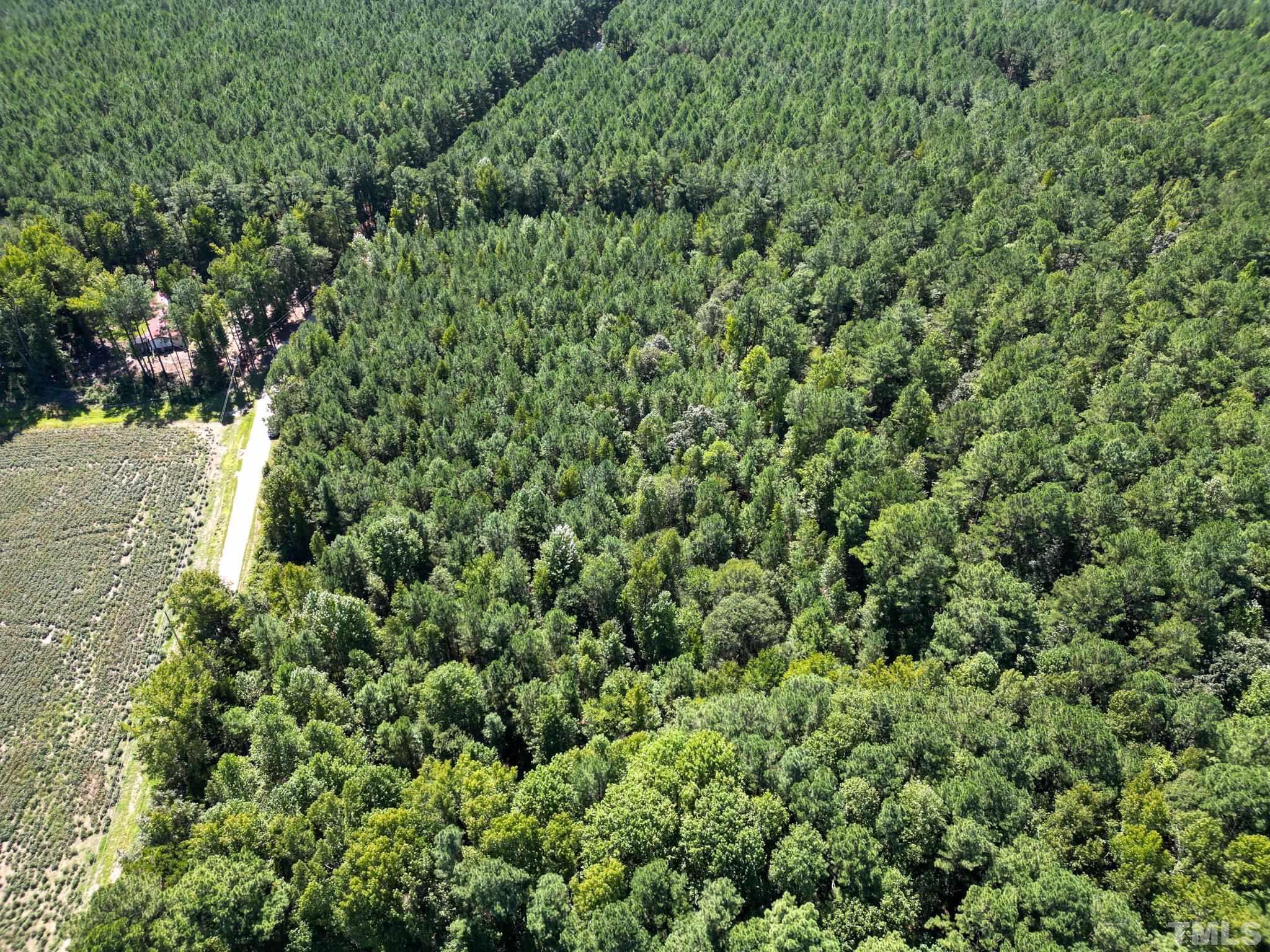This aerial image showcases a sprawling forested area dominated by a dense canopy of large, green deciduous trees, interspersed possibly with some evergreens. The extensive coverage of treetops occupies the majority of the frame, giving an impression of endless miles of verdant wilderness. Cutting through this thick forest, a small road meanders from the left-hand side, though it is partially obscured and disappears into the trees. Nestled within the woods, near the north of this road, stands a house distinguished by a reddish clay-colored roof and a white facade, almost hidden by the lush foliage surrounding it. In the bottom left corner of the image, there appears to be a section of farmland—characterized by what looks like rows of a small crop—adding a patch of lighter green to the predominantly dark green landscape. The scene is serene and devoid of human presence, creating an untouched and tranquil atmosphere.